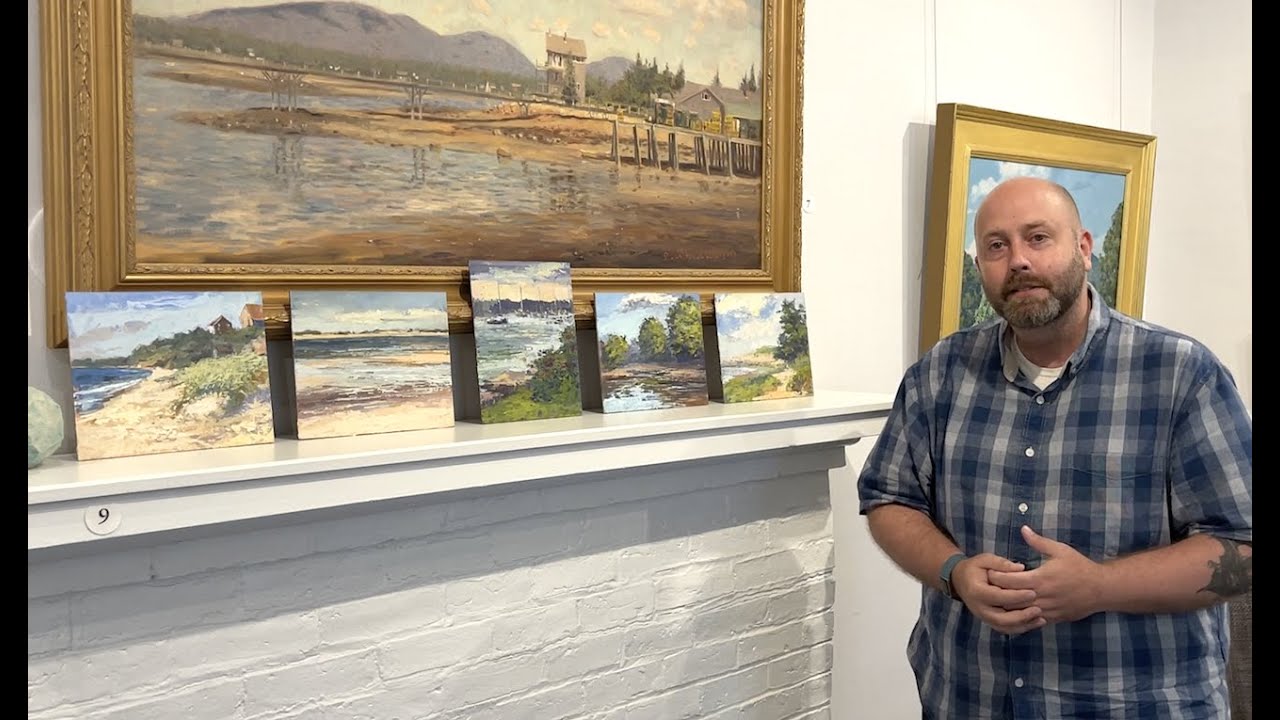In this horizontally rectangular, full-color photograph, a man is standing on the right side in front of a white-painted brick mantel that likely belongs to an older home. The mantel, which may be part of a fireplace not visible in the image, features a shelf displaying five small unframed paintings, each depicting serene beach and shore scenes. The mantel is flanked by several additional paintings, some hanging from frames and wires on the wall. The photograph itself has a thin black border running vertically along the left and right sides.

The man, visible from the waist up, sports a slightly open blue and grey plaid shirt over a white t-shirt and clasps his hands in front of him. He wears a blue wrist-banded wristwatch on his right wrist and has a noticeable tattoo on his right forearm. He is a balding gentleman with a full beard and his demeanor suggests a sense of pride, making it plausible that he could be the artist of the various seaside and forested lakeside artworks around him. The most prominent piece above the mantel is an ornately framed painting depicting a landscape with mountains, a dock, a beach, and water. His gaze is directed towards the camera, adding a personable touch to the image.